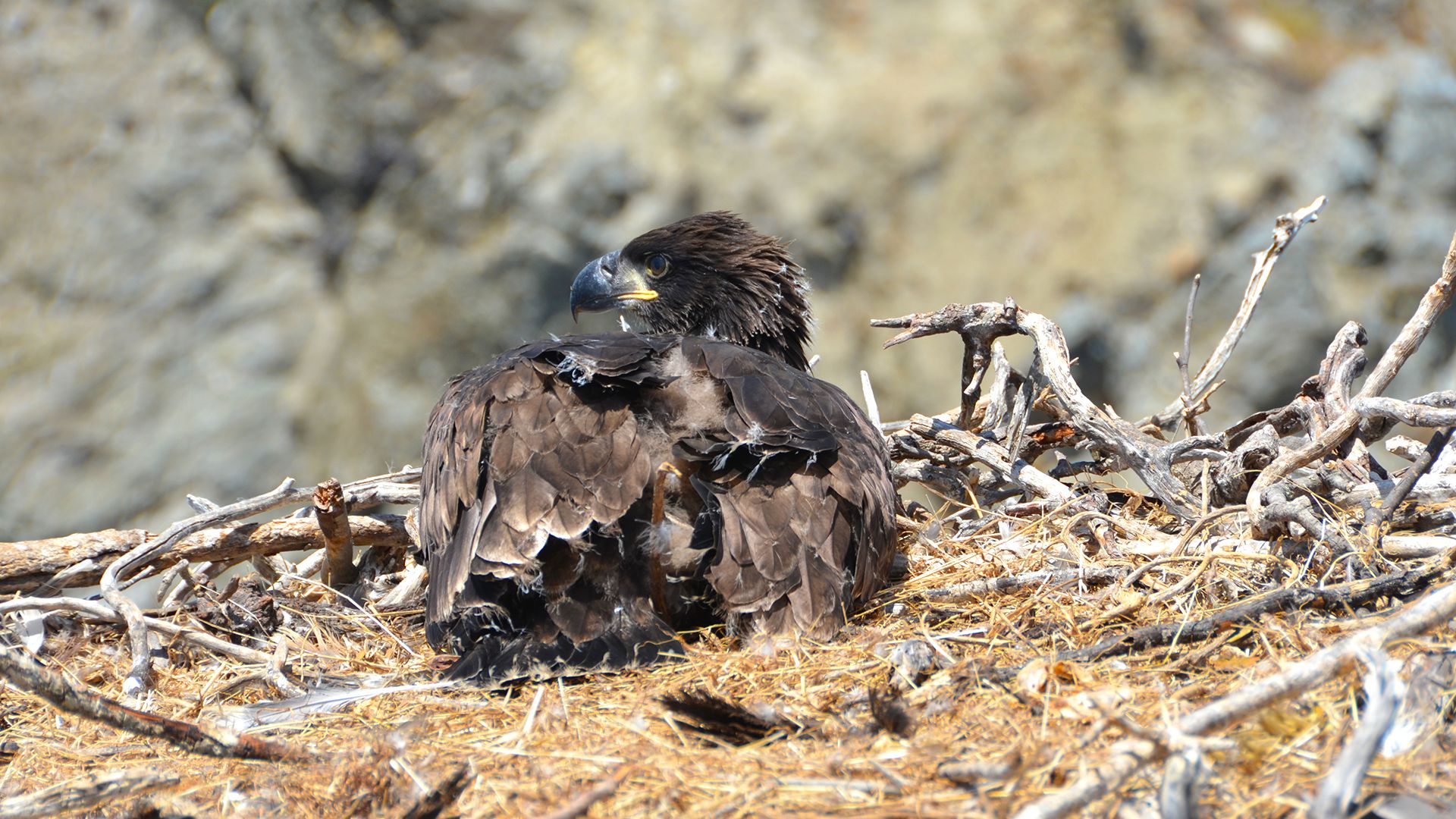This wildlife photograph captures a golden eagle in striking, bright, sunny light. Taken in close-up, horizontal orientation, it focuses on the back view of the eagle sitting on its elaborate nest, constructed from large twigs with smaller twigs in the center. The bird's head, covered in dark brown feathers, is turned to the left, revealing a sharply hooked beak that is black with a yellow hinged part near its eye. Its eye, encircled by a lighter ring, is brown and gazes intently at something off-camera. The eagle's plumage is predominantly brown with slightly lighter tips on the feathers. The background is intentionally blurred, suggesting a rocky cliff face or possibly more trees, contributing to the natural setting of the scene. The photograph is illuminated by direct sunlight, eliminating any shadows and highlighting the intricate details of the eagle and its nest.